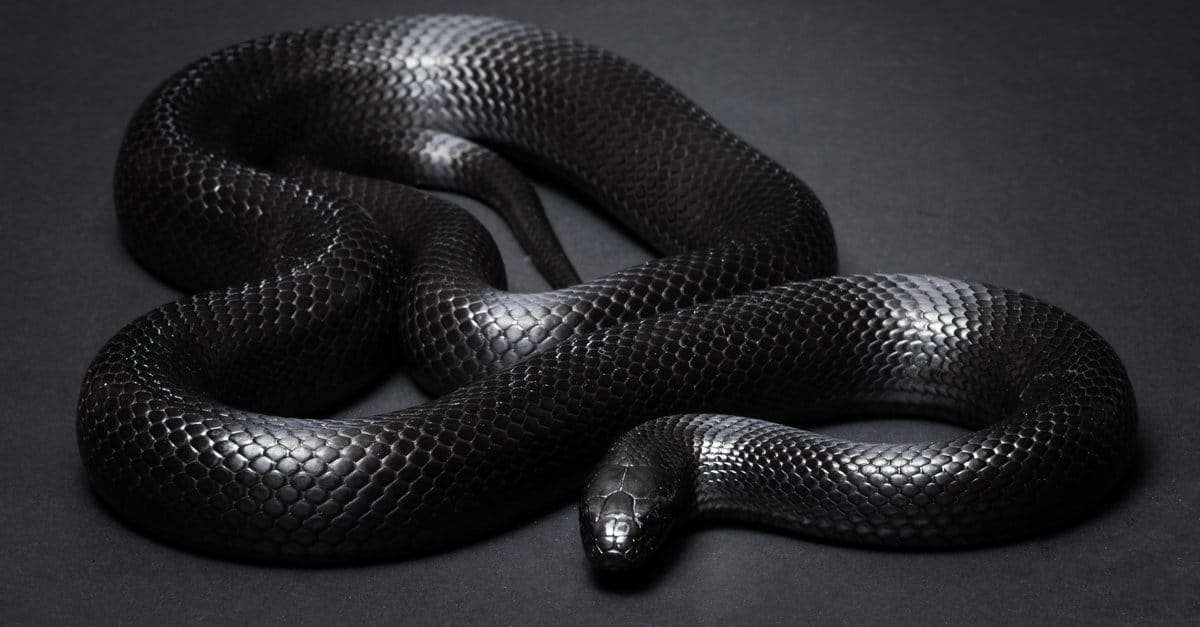This image features a striking, large black snake set against a matte black background. The snake, which appears to be approximately six feet in length, is prominently displayed in the foreground and fills most of the frame. Its glossy scales contrast with the matte surface beneath it, creating a dynamic visual effect enhanced by patches of light reflecting off its body.

The snake is coiled in a serpentine "S" shape, starting at the bottom of the image where its face is positioned and looking directly toward the camera. The body curves to the right near the edge of the frame, then sweeps across to the left and ascends toward the top. It continues curling back and forth, suggesting a loosely coiled figure-eight or heart-like shape before wrapping around to the right again and almost reaching the middle of the image.

The head of the snake is clearly visible and appears to be relatively calm, although its direct gaze gives an intense focus to the image. There is a shadow shading parts of the scene, adding an extra layer of depth, while the lighting causes the snake's smooth, small scales to glisten in places. Overall, the combination of the snake's impressive size, the sleekness of its shiny black body, and its poised posture makes for an intimidating yet mesmerizing photograph.